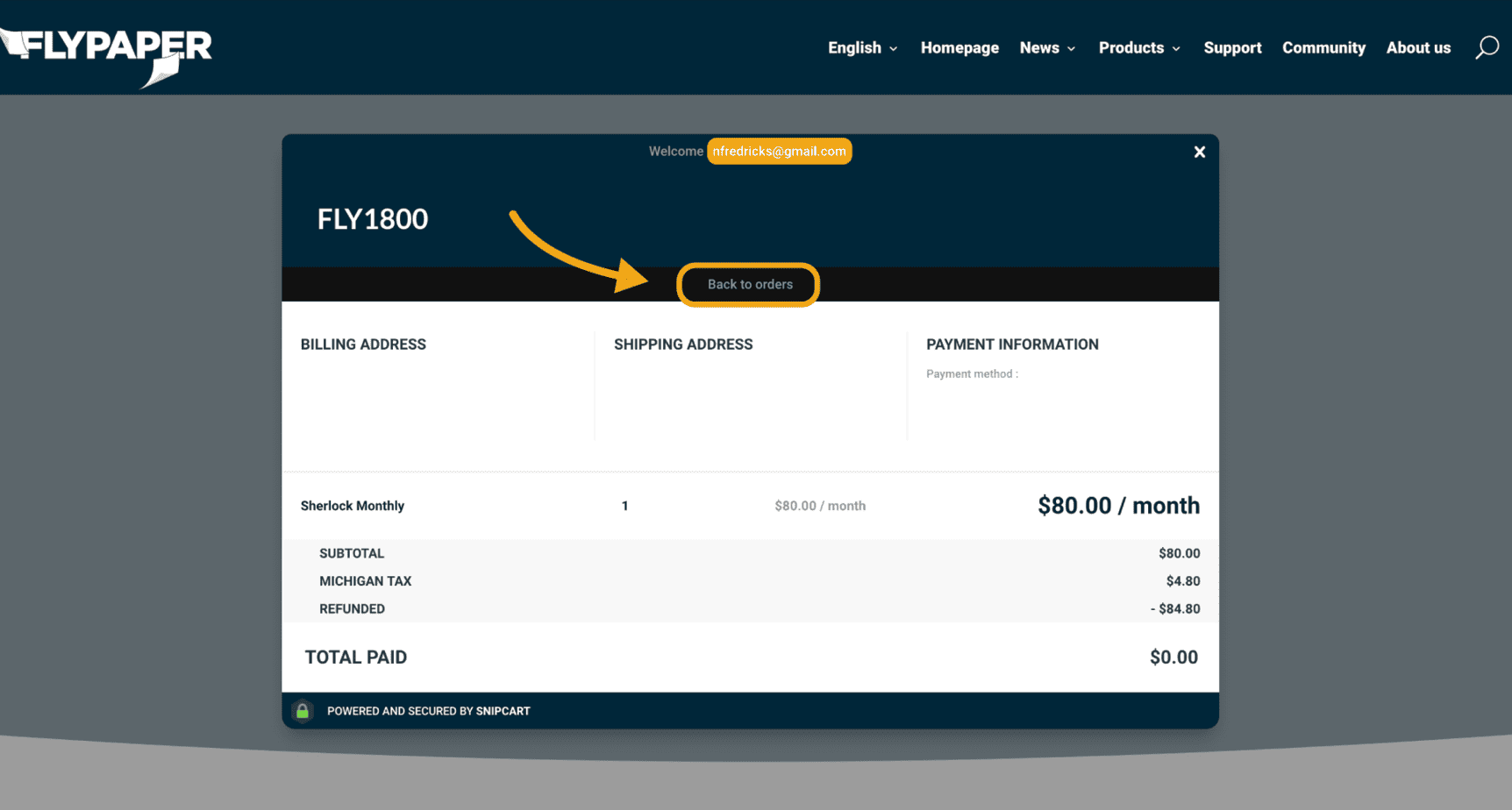The website features a sleek black navigation bar at the top, prominently displaying "Flypaper" on the left-hand side in crisp white text. Starting mid-way across the bar and extending to the right, there is a series of navigational links also in white text: "English," "Home Page," "News," "Products," "Support," "Community," "About Us," and an icon of a magnifying glass representing a search function.

The main content area has a dark gray background. Centrally positioned on this background is a large rectangular box. Inside this box, there is a label "Fly 1800" accompanied by an arrow. Below this is another white rectangle containing black text, with an orange arrow pointing toward a middle section that contains some unreadable words due to their small size.

At the bottom of the page, there is a light gray bar. Within the dark gray section above this bar, the text is white, standing out against the background. The white areas within the page feature black text for clear readability. Specific sections within the central box include "Billing Address," "Shipping Address," and "Payment Information." There is also a small "X" located at the top-right corner of this central box, presumably for closing or exiting the section. The finer details of the words within the box are too small to be discerned.